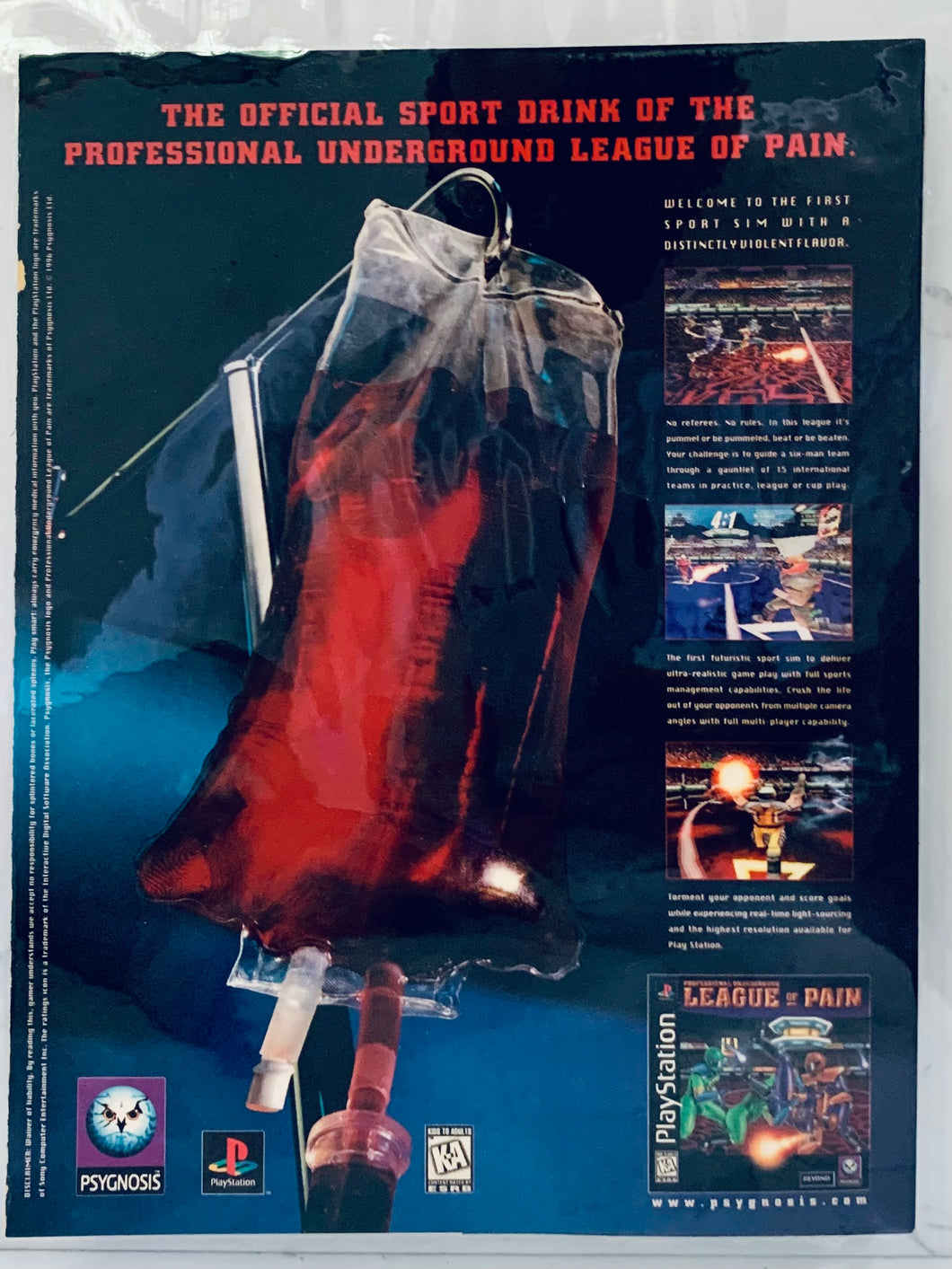The poster features a blood bag hanging from a silver IV pole, implying humor and violence to promote the PlayStation game "League of Pain." Set against a dark navy blue background, the top of the poster boldly declares in red letters, "The official sport drink of the Professional Underground League of Pain." Hanging from the pole, the clear plastic blood bag is almost entirely filled with a red liquid, with a tube extending from the bottom. On the right side of the image, the poster invites viewers with the text, "Welcome to the first sport sim with a distinctly violent flavor." Below this, four small images showcase gameplay scenes, each accompanied by a short, unreadable paragraph. In the bottom right corner, there's a small square showing the PlayStation game box for "League of Pain," marked with a K-A rating. Compact and somewhat difficult to read, additional text runs along the left edge of the poster.